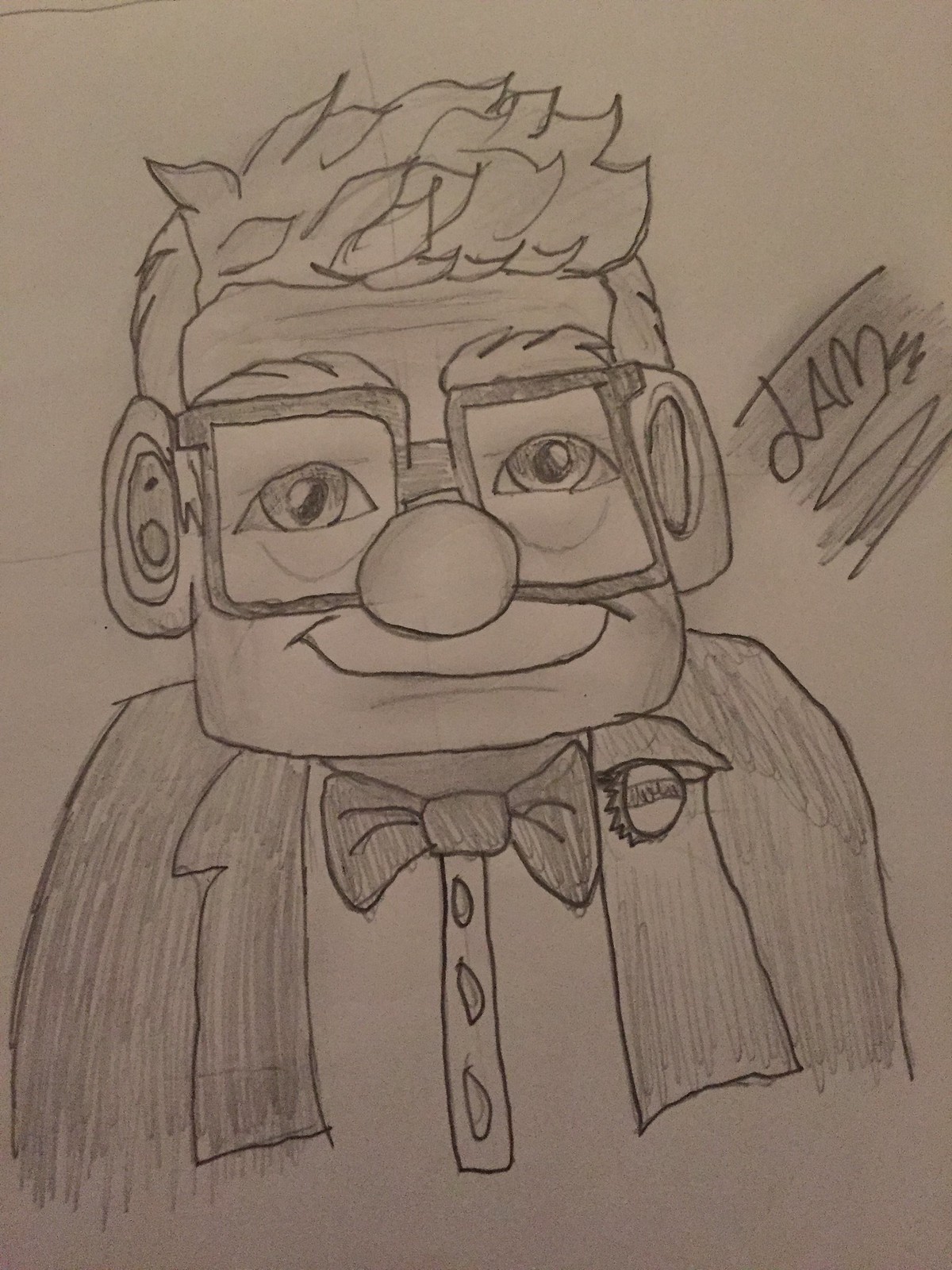This detailed pencil drawing, rendered on white paper, captures a character reminiscent of Carl Fredricksen from the movie "Up." The figure prominently features short, flowing hair and a distinctly square-shaped head complemented by fairly large ears. The character is adorned with squared-off glasses, which rest atop a prominent, round nose. A wide, toothless grin spreads across the character's face, adding to the cheerful expression.

The figure is dressed in what appears to be a tuxedo, complete with a bow tie. The tuxedo is depicted in an open position, revealing the buttons of the shirt underneath. Adding to the authenticity of the artwork, a signature from the artist is visible on the right side of the image. The attention to detail in this black-and-white sketch brings the beloved character to life in striking simplicity.